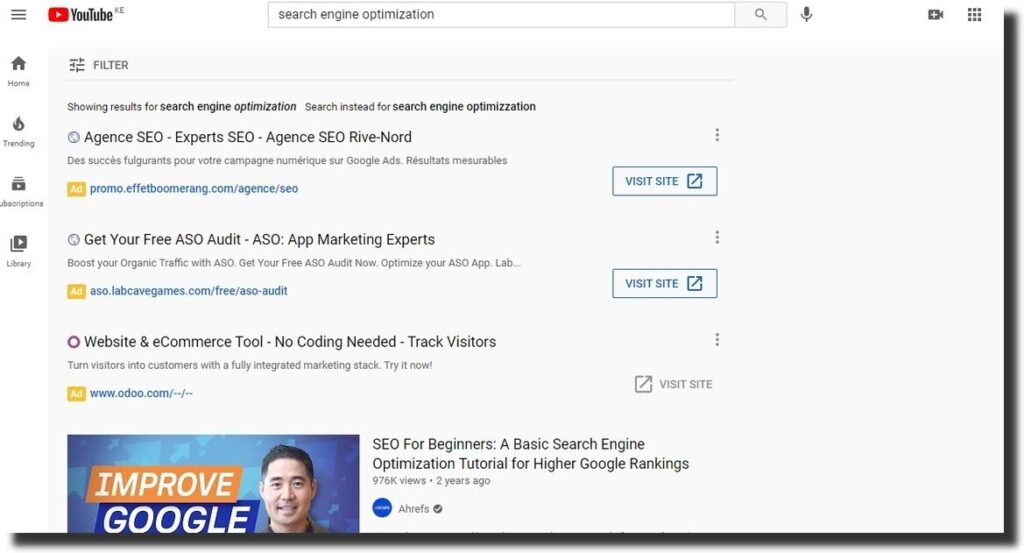Screenshot of a YouTube Search for "Search Engine Optimization"

In the screenshot, a YouTube search for "Search Engine Optimization" displays several results. The first result is partially obscured and seems to be in a foreign language but mentions agents and SEO experts. The second result reads "Get Your Free ASO Audit - ASO App Marketing Experts" with additional information and a link for further details. The third result is a tool for websites and e-commerce, described as requiring no coding and offering visitor tracking.

At the bottom of the screenshot, partially visible, is a thumbnail of a video titled "Improve Google," featuring a man apparently explaining the basics of SEO. The video's description states "SEO for Beginners: A Basic Search Engine Optimization Tutorial for Higher Google Rankings." This video has garnered 976,000 views and was uploaded two years ago. 

Overall, the search results provide a mix of SEO services, tutorials, and tools.